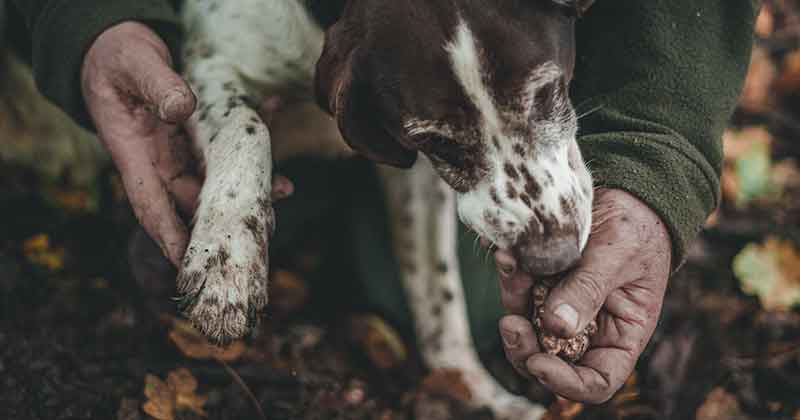In the image, a close-up captures a brown and white hound dog with distinctive markings; its head is mostly dark red-brown with a mixture of white and brown between its eyes, and a speckled white muzzle with brown spots. Centered in the frame, the dog eagerly reaches for food held in a man's dirty, crackled hand, which has dark spots and age marks. The man’s right hand lifts the dog's right paw, which is mostly white with brown speckles. The man wears a dark green fleece long-sleeved jacket. In the background, dark autumn leaves and dirt can be seen, adding a rustic touch to the scene.